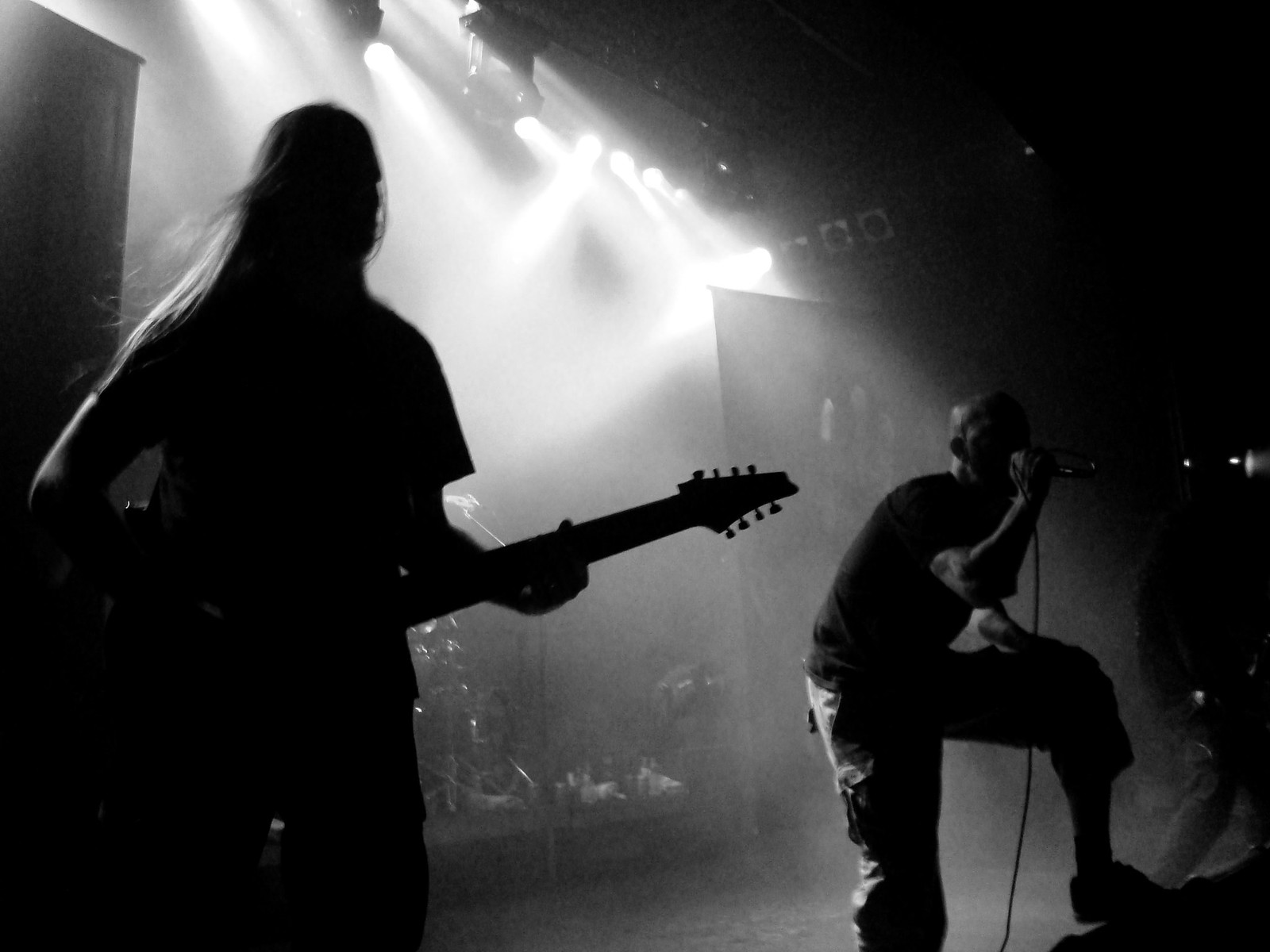In this captivating black and white landscape photograph, a dynamic rock band performs live on stage, illuminated dramatically by backlighting from overhead spotlights. The stage is mostly shrouded in darkness, with the intense lighting casting the band members into striking silhouettes. To the left, a tall, long-haired guitarist is fully engrossed in playing an 8-string electric guitar, his silhouette revealing the intricate details of his instrument. His face and body are obscured, contributing to the mystique of his performance.

Adjacent to him, the bald, muscular singer commands attention, crouching toward the audience with a fervent scream into his microphone. Clad in a black t-shirt and camouflaged shorts that extend slightly past his knees, his energetic posture suggests an explosive performance. 

In the smoky haze of the background, the barely visible drummer keeps the rhythm, their presence hinted at through the cymbals and parts of the drum set peeking through. Several lighting panels flank the stage, enhancing the dramatic and immersive atmosphere of the scene.

The image captures the raw intensity and energy of the rock and roll performance, viewed from the front row of an enraptured audience.